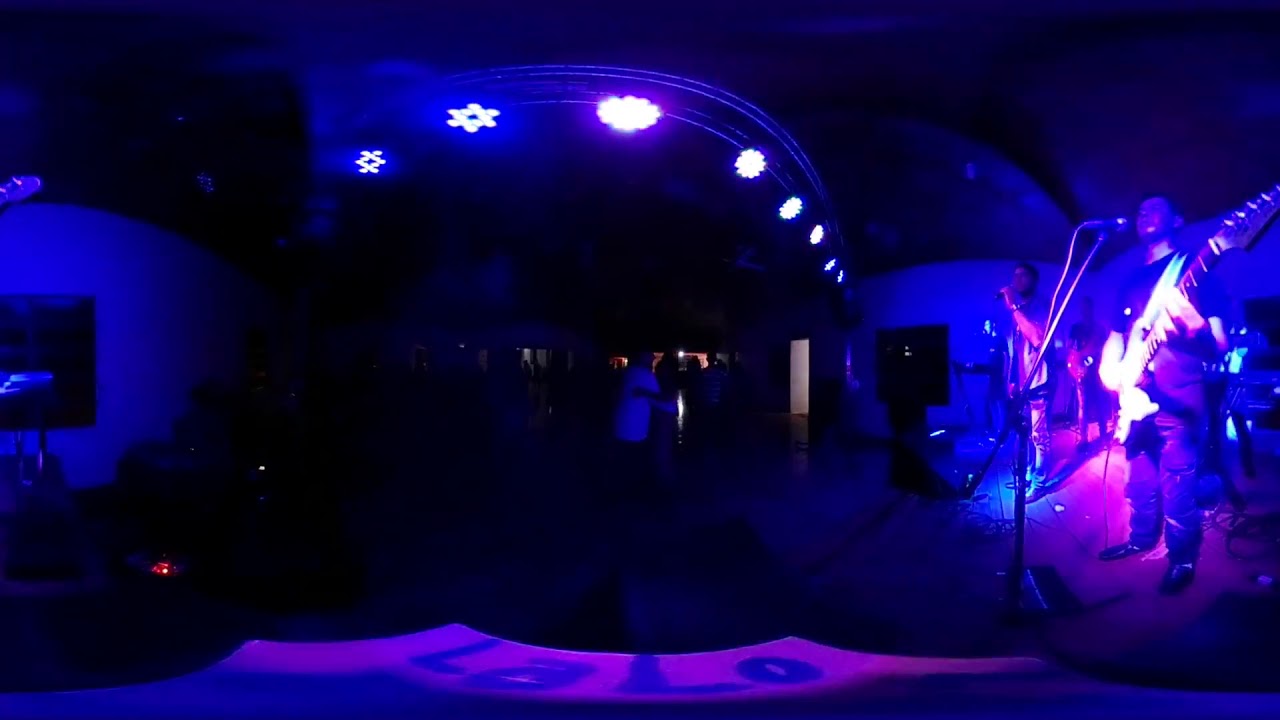In this vivid and dynamic landscape-oriented photograph, a band is captured in performance within a dimly-lit club setting. The image is composed as a panoramic view, merging three different angles to portray the scene comprehensively. Dominated by hues of purple, blue, and black, the stage is backlit, casting deep shadows and creating a visually striking backdrop.

To the far right of the image is the guitarist, prominently positioned under the brightest light, which bathes him in a blend of blue and purple. His shadow, tinged with a blue effect, extends behind him. Just to his left stands a microphone and its stand. Slightly obscured behind this setup is the lead singer, holding a microphone and glancing towards the center of the photograph. The singer's outfit, likely a t-shirt and pants, is difficult to discern due to the heavy shadows.

In the background, another band member is faintly visible, enveloped in a hazy purple light that obscures their details. At the right edge of the composition, partially covered by the guitarist, there appears to be an electric keyboard or another instrument setup.

The center of the image is notably dark, save for several overhead fixtures—approximately six or seven lights—casting their purple glow onto the band. This row of lights includes various shapes, contributing to the visual complexity. 

Beneath the stage, in the heavy shadows, a small crowd can be detected, their forms indistinct but suggesting a few spectators immersed in the performance. The photograph also features a lavender light at the bottom center, with the word "L-A-L-O" inscribed in blue, adding an additional layer of detail to the scene. The style of the image is photographic representationalism, enhanced by the panoramic filter that seamlessly blends the three images into one cohesive narrative.